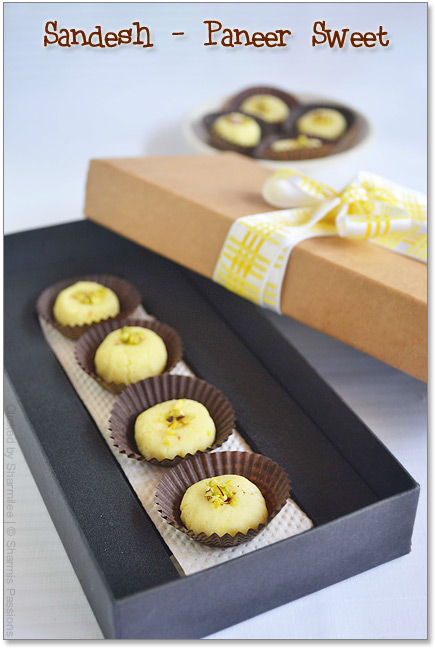The image is a professionally staged advertisement for a delectable bakery treat, elegantly presented in a rectangular dark green gift box with a tan, open top. The box features a white ribbon with yellow stripes, neatly tied into a bow. Inside, four round, cream-colored sweets, assumed to be "banana tips" or "sandesh dash paneer sweets," are meticulously lined up in dark brown paper wrappers reminiscent of those for Reese's cups. The background of the image is a soothing light blue with a slightly blurred depiction of the same treats arranged in a circle on a white dish. Prominently displayed at the top of the image in brown text is the label "Sandesh Dash Paneer Sweet." The entire setup is viewed from an upright angle, highlighting the elegance and detail of the presentation.